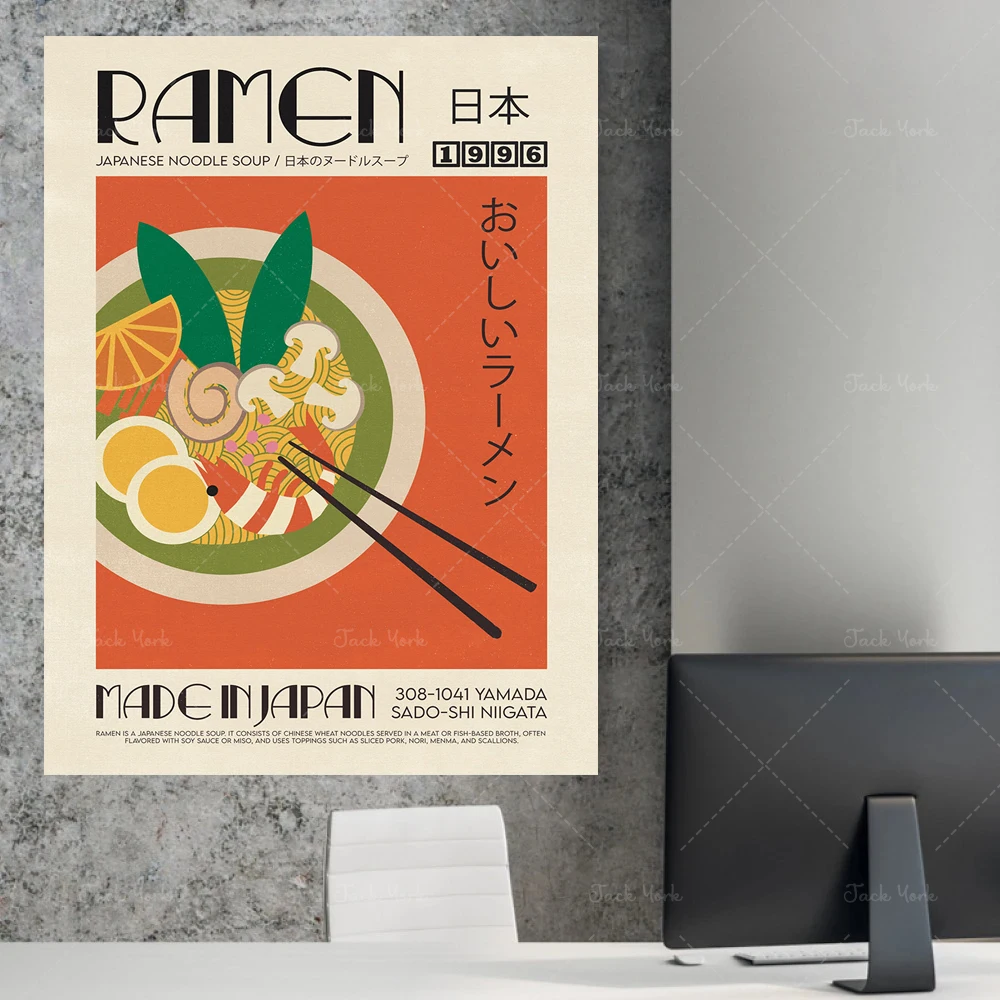The image depicts an indoor setting featuring a two-toned wall; the left side is covered in varying shades of speckled grey marble, while the right side abruptly transitions into a light grey segment adorned with a pattern of thin white dotted lines. Dominating the left wall is a poster with a thick beige border, showcasing an illustration of a bowl filled with ramen, shrimp, eggs, leaves, and mushrooms against a bright orange background. The top of the poster reads "ramen" in fancy black letters, followed by "Japanese noodle soup" in smaller print. There is additional text in Japanese on the right, along with the phrases "Made in Japan," "1996," and "308-1041 Yamada S-A-D-O-S-H-I-N-I-G-A-T-A" written in black. At the bottom of the image is a white table with a darker grey desktop computer partially visible alongside a white chair. Overlaying the entire image is a watermark consisting of diagonal dotted lines with the text "Jack your pay."